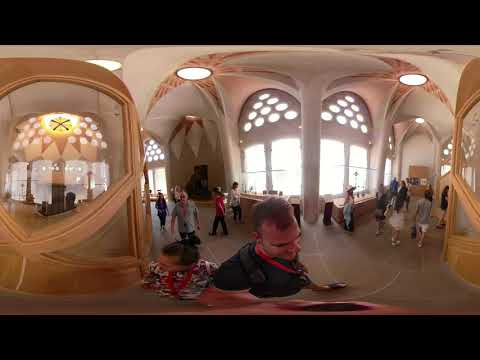This picture captures a bustling hallway within a large and brightly lit entryway of what appears to be a tourist hotel, illuminated by daylight streaming through numerous arched windows featuring circular designs. Tourists are scattered throughout, traversing two separate walkways that lead in different directions. At the forefront is a younger man in a black t-shirt and shorts, adorned with a red bandana or tag around his neck, accompanied by a shorter woman in a floral blouse. To their side, another man in his 60s with sunglasses approaches. The scene is populated with many individuals, some of whose distorted arms can be observed due to the camera's perspective. White lights adorn the ceiling, which is supported by three visible columns and showcases a distinctive triangular window at the top.